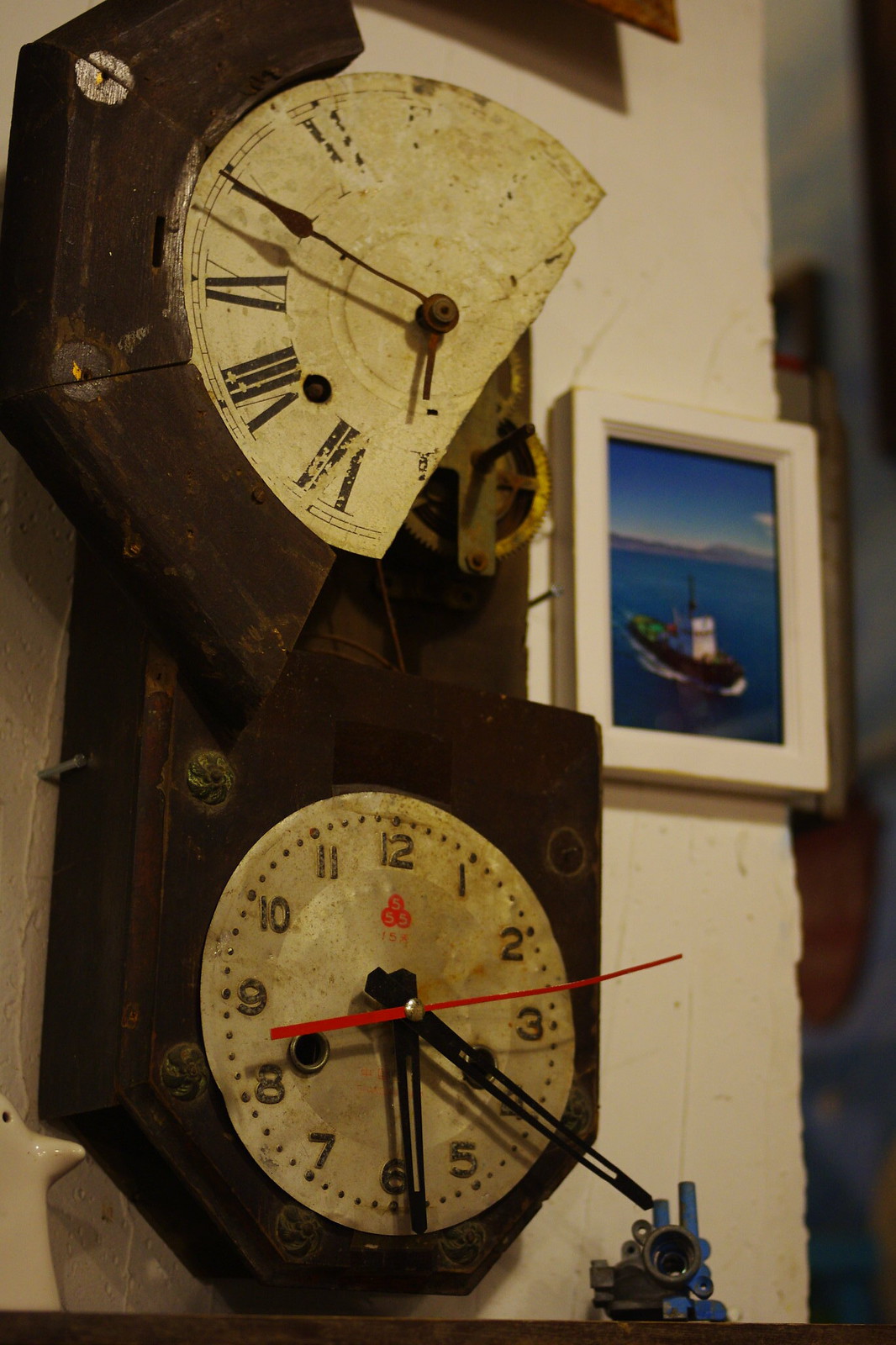The photograph depicts a rough, white, and somewhat dilapidated wall adorned with two old clocks and a framed painting. On the left side of the image, the focal point is two clocks. The upper clock is notably damaged, with its top portion broken off, exposing some internal gears and pulleys. This clock features a dingy, dusty face with Roman numerals, one of which is cut, revealing parts of the clock's wooden frame around the faceplate. The bottom clock is intact but aged, with a bright red second hand, black hour and minute hands, mounted on a wooden base and surrounded by a white clock mount. 

On the right-hand side, there's a painting in a white frame that slightly extends off the edge of the wall. The painting depicts a small boat on a blue sea, adding a dash of color to the otherwise muted scene. Below and to the right of the clocks, there's the corner of another picture frame visible, casting a shadow on the upper part of the wall. Additionally, a metallic object, possibly a sculpture, is seen in the lower right corner of the image. The background spills into a blurred hallway, giving depth and context to the scene.